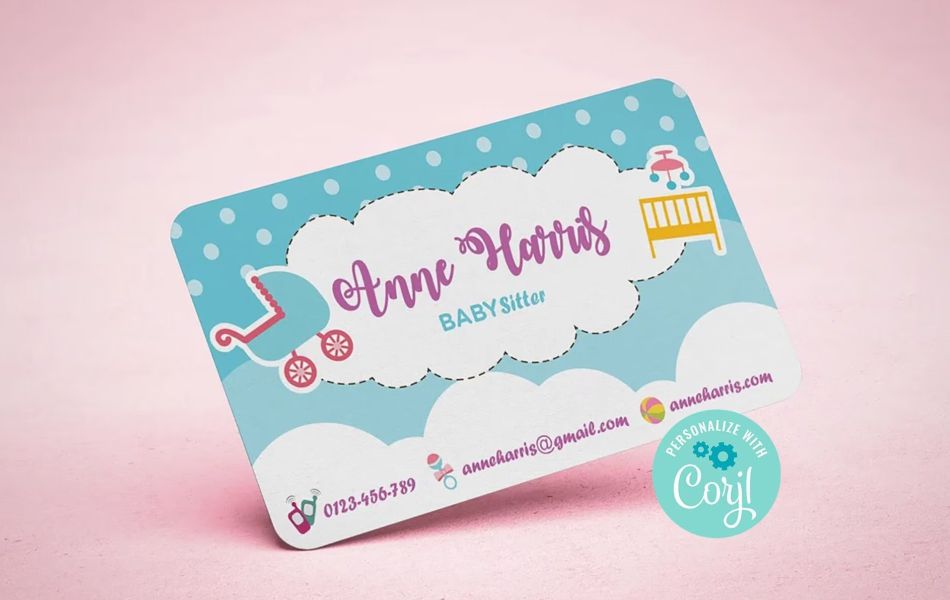The image showcases a stylized business card balanced on its left corner, set against a pink-purple background with a visible shadow beneath. The business card itself features a baby blue background accented with three rows of white dots at the top. In the center, purple cursive text spells "Ann Harris," followed by "Babysitter" in blue print, all elegantly placed within a fluffy, white cloud outlined in black dots. The left side of the card displays a blue baby carriage with red accents and wheels, while the right side features a yellow crib adorned with a pink mobile and blue balls.

At the bottom left corner, two cell phone icons precede a placeholder number: "012-345-6789." Adjacent to this is an email address, "annharris@gmail.com," and a website, "annharris.com." A baby rattle and colorful ball appear to the right of this information. The lower right corner of the image contains a blue circle with white text reading, "Personalized with Coriel!" emphasizing that this is a template design.